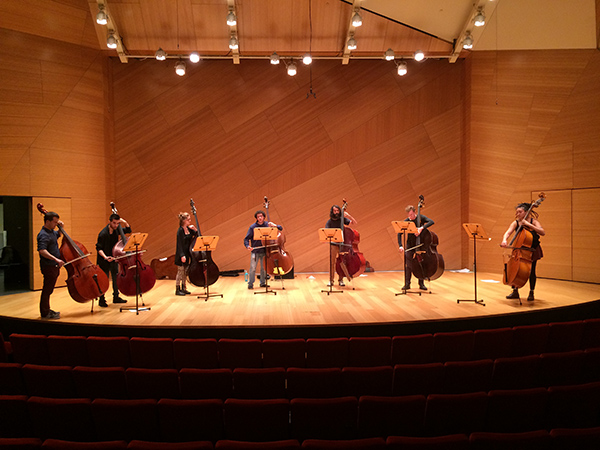This indoor photograph captures a performance by seven musicians on stage. They are arranged in a semi-circle, each with a cello and a music stand in front of them. The stage is made of light-colored wood, with matching wood-paneled walls and ceiling. Bright studio lights from above illuminate the scene. The musicians appear to be a mixed group of men and women, dressed in various clothing. In front of the stage, you can see a black lower stage face and rows of maroon theater seats extending from the left to the right and partially visible at the bottom of the image. On the left side of the stage, there is an open doorway, while the right side features closed doors. The overall ambiance highlights the warm hues of the wood and the focused lighting on the performers.